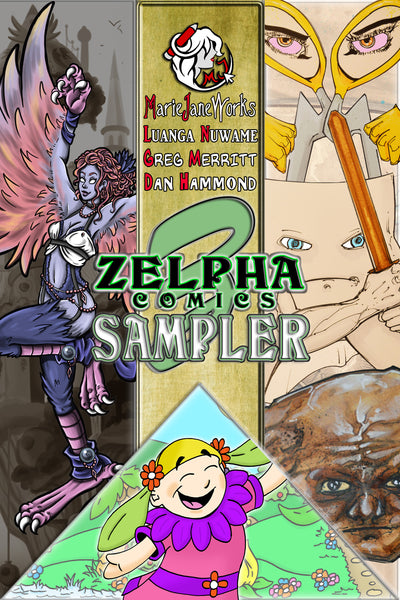This is an image of the cover of the comic book "Zelfa Comics Sampler Number Three." At the top, the cover lists the authors: Marie Jane Works, Luanga Nuwame, Greg Merritt, and Dan Hammond. The cover features a collage of distinct and imaginative artworks. On the left side, there's a fantasy illustration of a fairy-like woman with bird-like features—claw feet and hands, wings, and curly hair with white eyes, dressed in purple. Another prominent image showcases a woman peering through a pair of scissors. There is also a surreal portrayal of a torso with a face holding a sword. Additionally, there's a bizarre figure resembling a brown blob man. At the bottom, a whimsical cartoon depicts a little girl running through a forest, laughing and wearing a pink and purple dress with flowers adorning her pigtails. Other details show her with flowers around her neck and leaves for hair. The center of the cover prominently displays the title "Zelfa Comics Sampler."